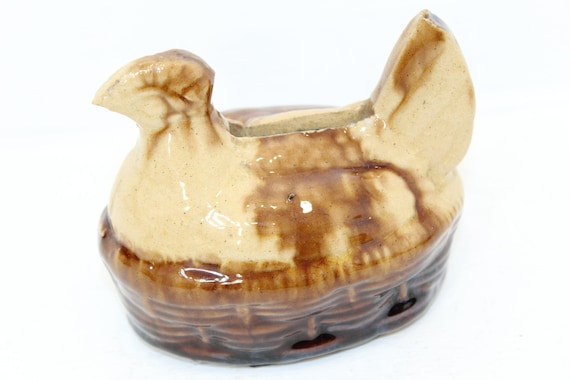The image features a small, shiny ceramic item against a white background. The item is shaped like a hen sitting in a woven basket. The top part of the hen is glazed in a light beige color, with darker brown accents on the tail and head. The bottom part of the ceramic hen, which is designed to resemble a woven basket, is glazed in a darker brown. Additionally, there is a slot on the top back of the hen, indicating that it functions as a piggy bank.